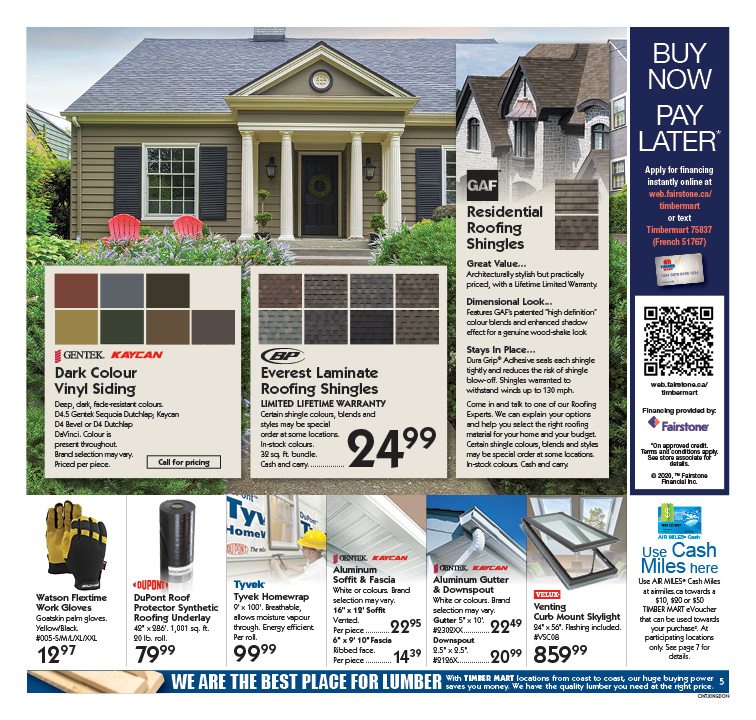In this image, we see a physical advertisement, likely cut from a newspaper, that focuses on home improvement items. The top of the ad showcases a picture of a charming house, setting the theme for the various products displayed below. 

On the left side, there's an advertisement for dark-colored vinyl siding, available in several shades, visually represented just to the right. Adjacent to this, another section features Everest laminate roofing shingles, boasting a limited lifetime warranty, priced at $24.99 each with examples of the shingles provided.

Continuing to the right, the ad lists different types of residential roofing shingles with detailed descriptions. The bottom section of the advertisement highlights an array of essential home improvement items, including work gloves, roof protectors, home wrap, aluminum siding, gutters, and various venting products.

Additionally, on the far right, there is a promotion for a special financing offer — a card that allows customers to "Buy Now, Pay Later," giving a convenient purchasing option for the customers.